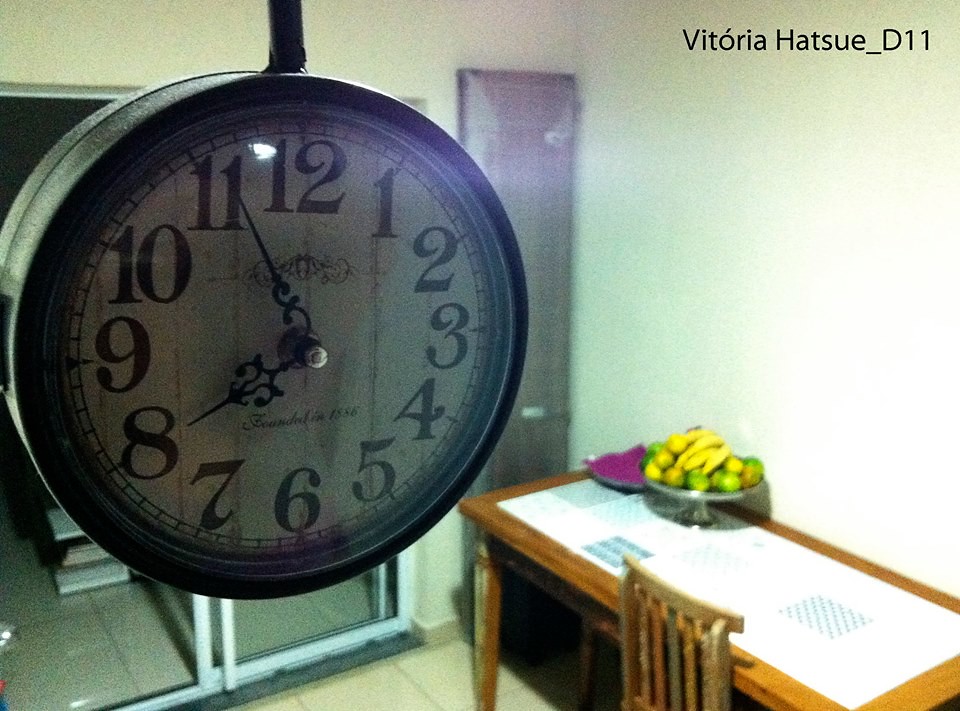The image depicts a wooden desk or table with a matching wooden chair, covered by a large sheet of white paper, situated in a room with beige tile floors. A silver tray adorned with a variety of fruits including bananas and limes rests on the desk. The room evokes the feel of a classroom or a police precinct, as suggested by the overall setting. Dominating the scene is a round wall clock, intricately designed with ornate hands and large, stylized numbers 1 through 12. This clock, encased in a thick black frame with a white face and an antique appearance, is suspended from a thin black bar descending from the ceiling. The clock seems to display a time near either 11:40 or 7:55, partially obscured by a greenish tint. The background is further detailed with a folded table in one corner and a sliding glass door on the left. Upper right-hand text reads "VITORIA HATSUA underscore D11."